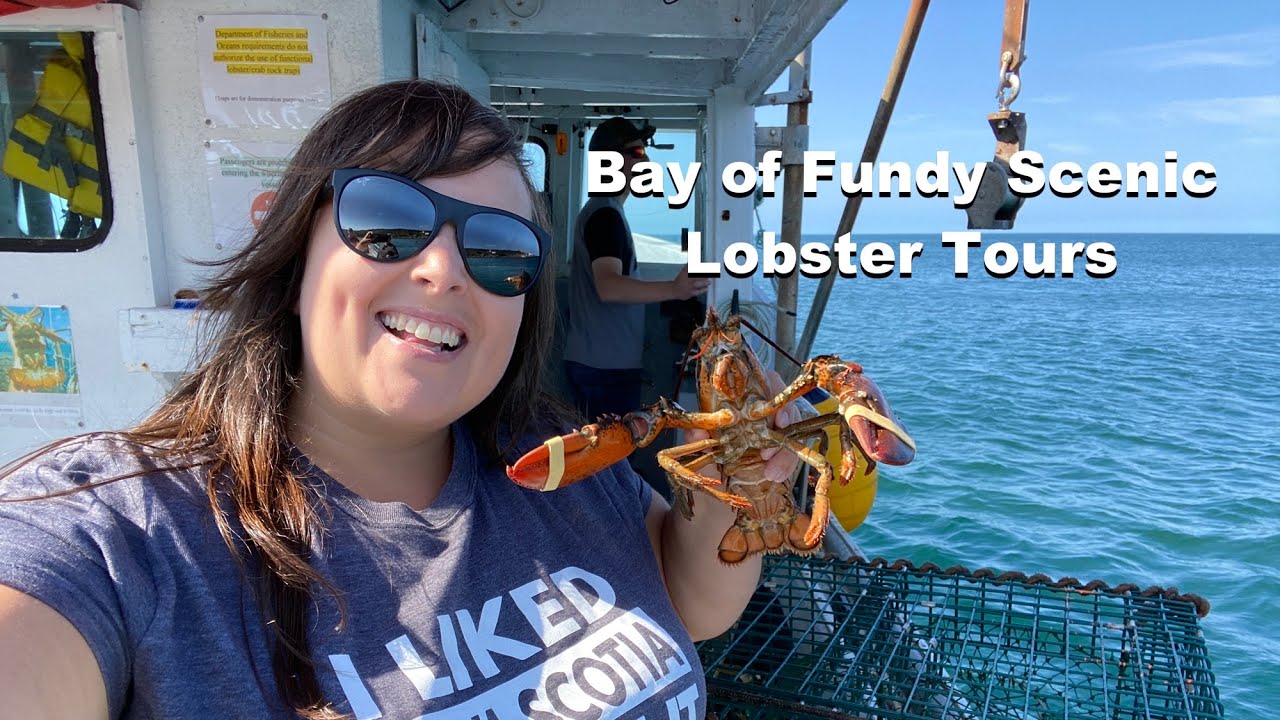In this horizontal rectangular photograph, an advertisement for a business, a woman appears on a lobster boat amidst choppy waters under a mostly blue sky with sparse clouds. Holding a small lobster with rubber-banded claws, she wears sunglasses and smiles warmly. Her long dark hair cascades over her shoulders, and she sports a blue-purple t-shirt with partially visible text that reads "I liked Nova Scotia". The woman stands near a lobster trap on the boat's deck, with the white-walled cabin and its pillars visible behind her. A person, presumably the captain, is seen steering the boat. Prominent white text in the upper right corner reads, Bay of Fundy Scenic Lobster Tours, cementing the image as an enticing advertisement for the scenic aquatic adventure.